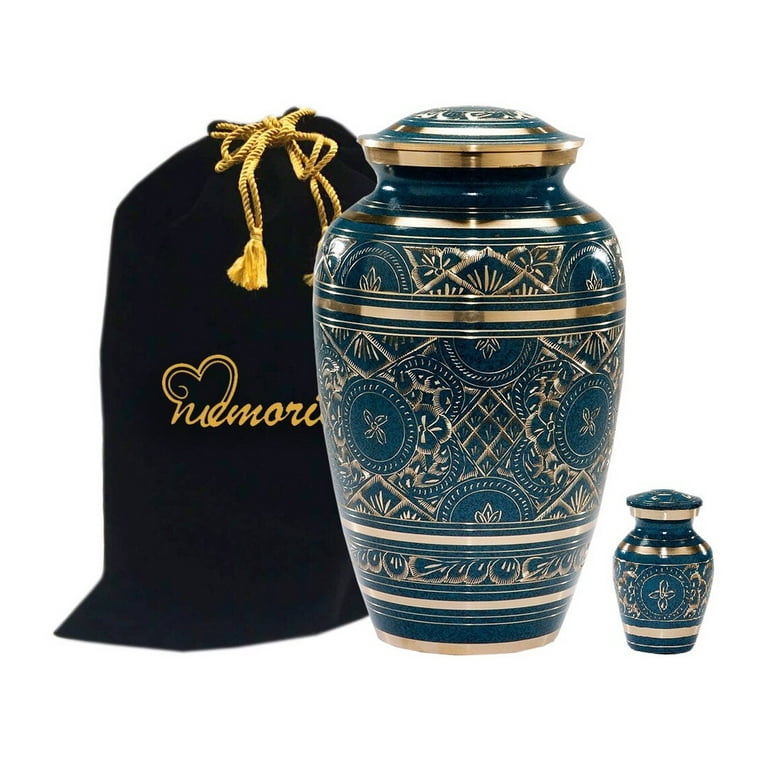This image appears to be a graphic design with no background, showcasing two ornate, blue teal urns and a storage bag. On the right side is a very small urn adorned with intricate gold ornate patterns and a round, teal lid featuring white trim. This small urn starts narrow, widens slightly toward the top, and is approximately one-fourth to one-fifth the size of the larger urn to its left.

The larger urn is similarly designed, with the same blue teal hue and gold ornate designs, but includes gold trimming on its round lid. This large urn is prominent with a more robust Middle Eastern-inspired design, featuring three deep gold lines and an expansive gold pattern detailing near the top and bottom.

Partially hidden behind the large urn is a black velvet bag tied with a gold rope fashioned into a bow. The bag appears to have cursive gold text across the center, partially obscured by the larger urn. The image captures the elegance and ornate details of these memorial urns against a white background.